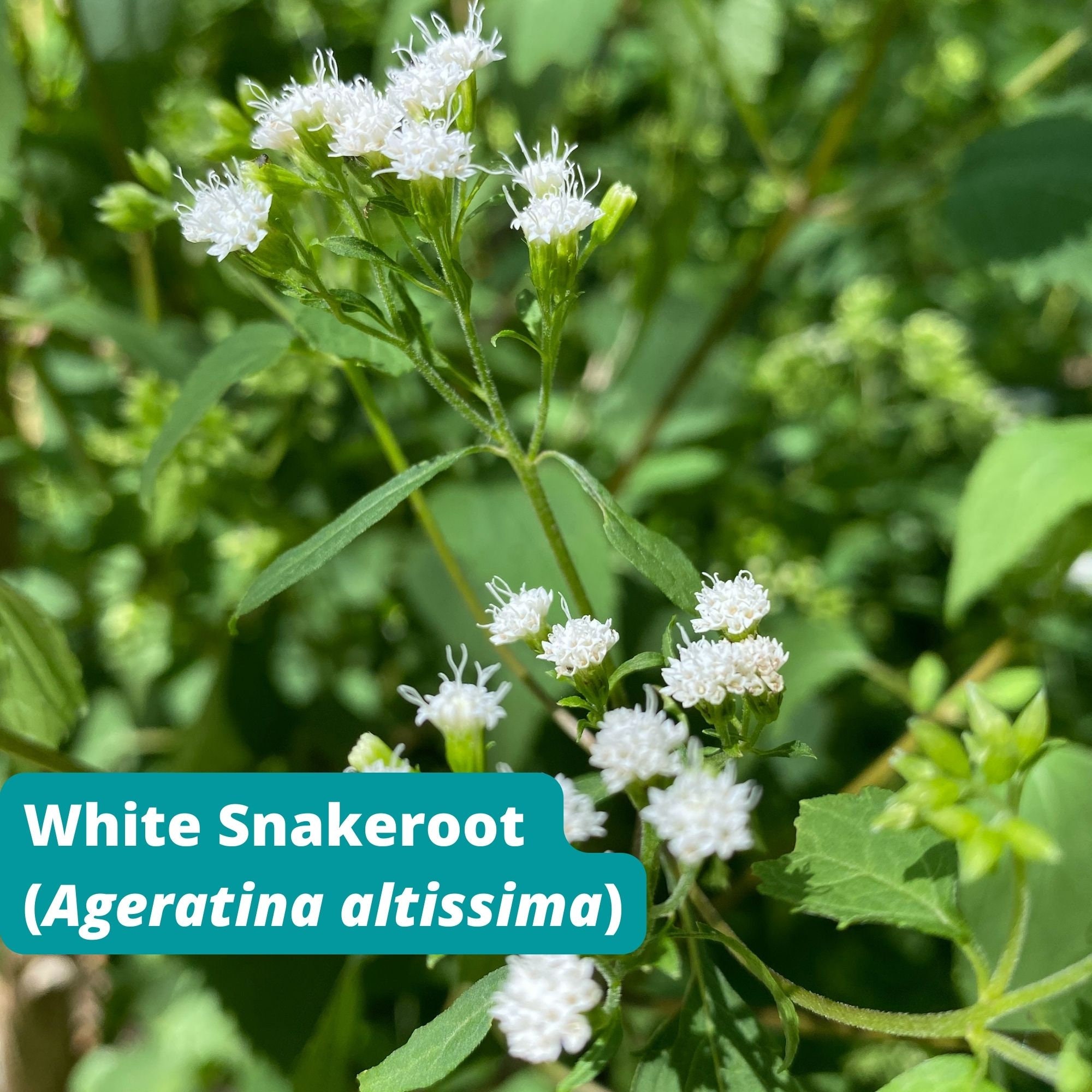This square image captures a detailed view of a plant known as White Snake Root (Agaratina altissima). Dominating the scene are clusters of small, delicate, white, fibrous flowers with wavy, noodle-like appearances. These flowers, which form roundish bursts at the end of slender green stems, are scattered throughout the image, appearing both at the center top and bottom middle sections. The plant's leaves, varying in size and hues of green, create a verdant, albeit blurry, backdrop. In the lower left corner, a teal box with white text designates the plant's common name, "White Snake Root," followed by its scientific name, "Agaratina altissima," in parentheses. Overall, the composition accentuates the intricate floral details against a lush green setting, possibly indicating its source as an informational magazine or book entry.